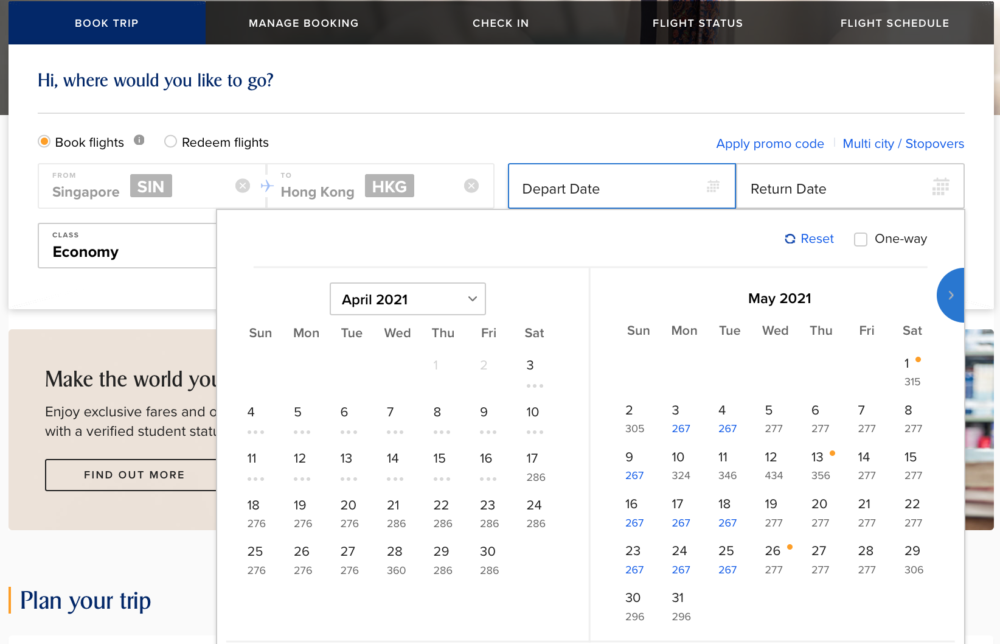**Detailed Caption:**

The image displays a webpage from a flight booking company. The top section features a header with a navigation menu. The first item on the left, "Book Trip," is highlighted in dark blue, indicating it is the currently active selection. The rest of the menu items, "Manage Booking," "Check In," "Flight Status," and "Flight Schedule," are in black.

Below the header, the main content area has a white background. In the top-left corner, there is a welcoming message that reads, "Hi, where would you like to go?" Below this greeting, a light gray horizontal line separates the sections. Under the line, a highlighted orange circle indicates the "Book Flights" option, flanked by an inactive gray circle to its right and an inactive white circle further to the right, representing other booking options. Next to this selection is the option "Redeem Flights."

Below these selections, the booking interface appears. There are several input boxes for flight details. The first box, labeled "Singapore," contains the airport code "SIN" inside a gray box. To its right, the next box is labeled "Hong Kong" with the airport code "HKG" in a gray box. Further to the right, there is a "Depart Date" box highlighted with a blue border, indicating it is the active field. The depart date box opens a calendar display showing the months of April 2021 on the left and May 2021 on the right. Each date on the calendar has a price listed underneath, indicating the cost of the flight ticket for that specific day.